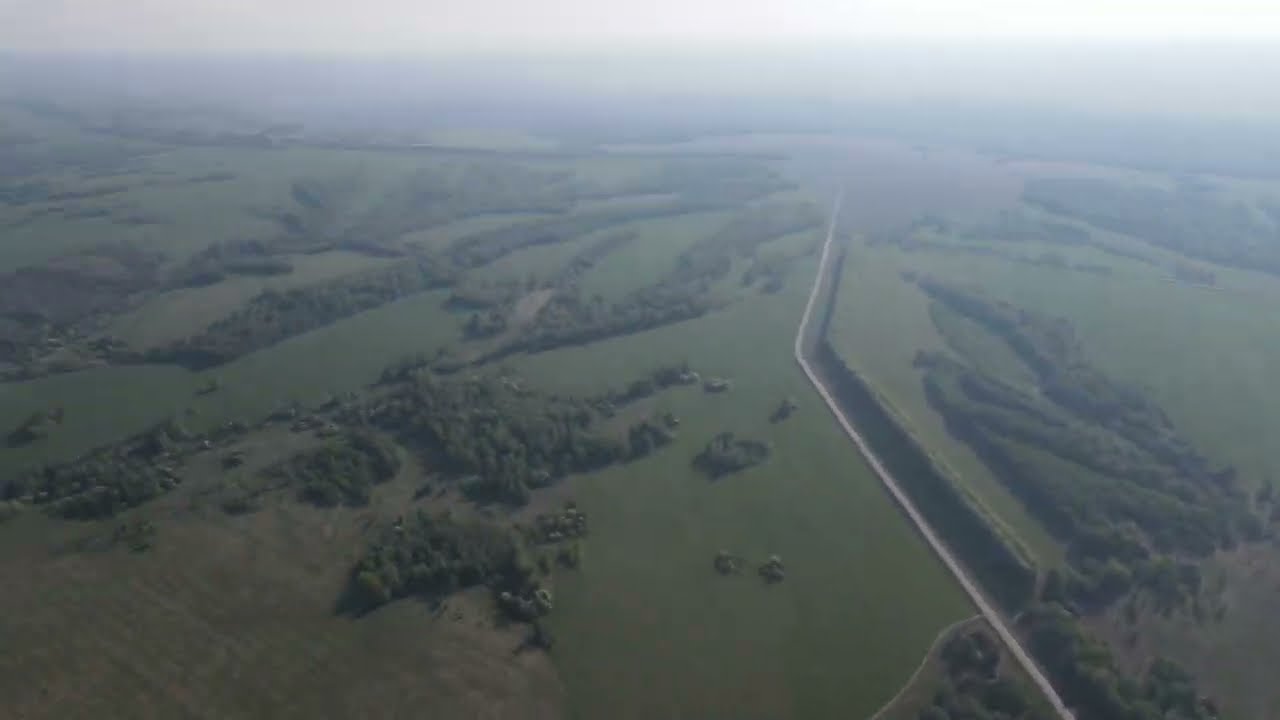This aerial color photograph, measuring 8 inches wide by 5 inches tall, captures a vast, lush green landscape, suggesting it was taken from either an airplane window, helicopter, or drone. Dominating the scenery are expansive fields crisscrossed by well-defined man-made canals and property lines. Dense clumps of forest or heavy bush areas punctuate the wide-open spaces, giving a stark contrast to the grassy fields. A road enters from the bottom right corner, curves midway, and then veers off to the right, disappearing into the hazy distance. Toward the right side of the image, a significant water body, possibly a large lake or part of the River Everett, is visible. Tributaries and smaller channels emanate from this water body, weaving across the landscape. The background is marked by mist or natural haze, obscuring details and merging into gray mountains under a foggy sky above. The overall image quality is medium, with a photographic realism and representational style emphasized by the scattered light and soft, muted tones.